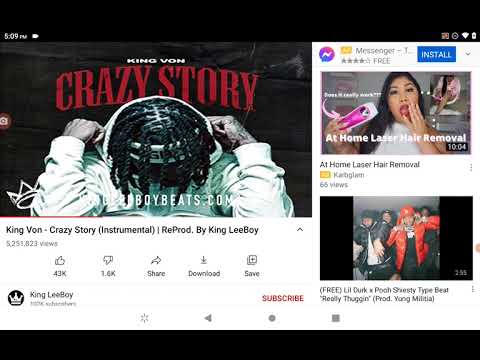This screenshot, captured from an internet webpage, showcases an instrumental track with several advertisements on the right side. At the top of the page, the timestamp reads 5:09 p.m. The track playing is titled "Crazy Story (Instrumental)" by King Von, reproduced by King Lee Boy. The associated image for the song features an African male with braided hair, his head slightly bowed. He is dressed in a white hoodie, partially covering a bandana or headband, and his face remains partially visible. The video has garnered 5,253,823 views, with 43k likes and 1.6k dislikes. Below the video, there are interactive icons: a thumbs-up for likes, a thumbs-down for dislikes, a share button represented by an arrow pointing right, a download button with a line and arrow, and a save button depicted as a square with a plus sign. The uploader's name, King Lee Boy, is displayed alongside a profile picture of a black circle featuring a white crown, and a prominent red subscribe button is centered below it.

On the right side of the screen, an advertisement for at-home laser hair removal is visible, featuring an Asian woman holding a pinkish rectangular laser device. Another section mentions "Free Lil Durk and Pooh Shiesty Type Beat - Really Fuggin Produced" by Young Matilda, with a blurred image of several African-American men wearing jackets and hats.